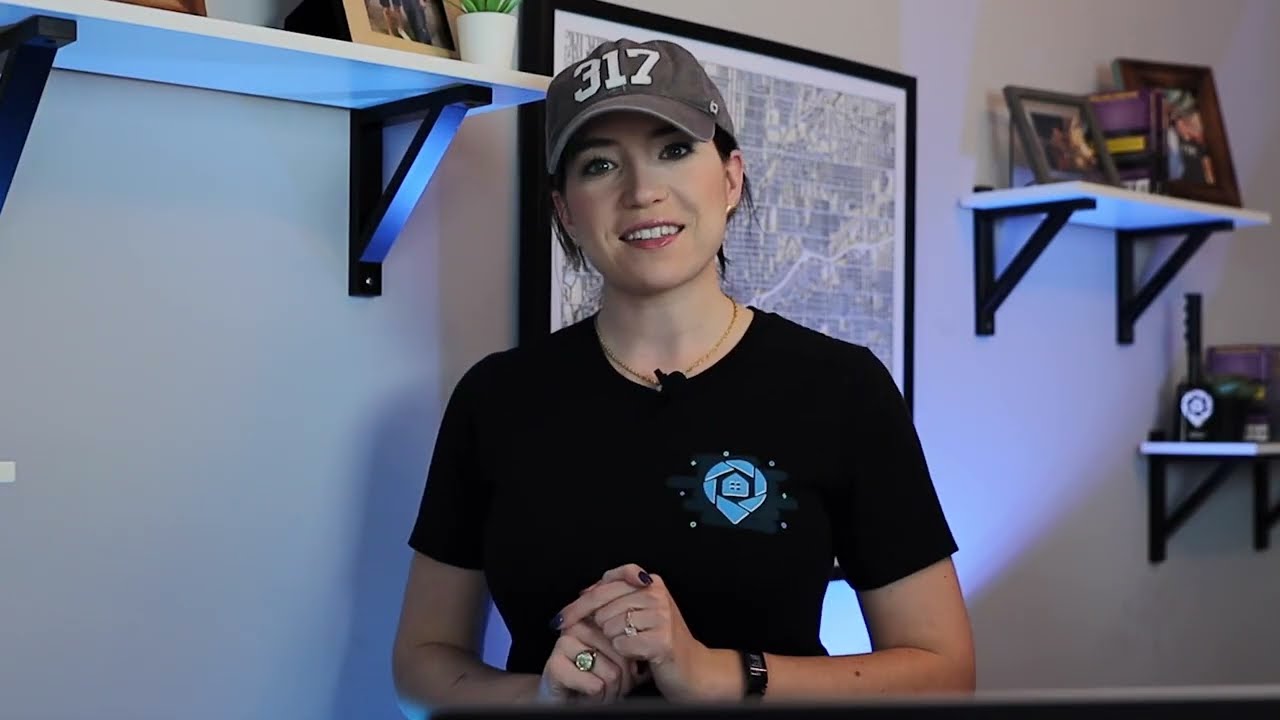The image captures a young woman in her mid-twenties with light skin, looking at the camera with a warm smile. She is wearing a gray baseball cap featuring the white numbers "317" and a black short sleeve shirt adorned with a blue logo, which consists of a circular design with a house in the center surrounded by dots. Her hair is pulled back, and she has a wristwatch on her left wrist along with rings on her fingers. She holds her hands in front of her, possibly preparing to speak, as a microphone is noticeable. The background reveals a clean, well-lit room with a white wall adorned with three shelves. These shelves hold a variety of items, including picture frames, books, and a small plant. There's also a large portrait that resembles a bird's-eye view of streets or a map. The setting suggests she might be giving a presentation or recording content for an audience.